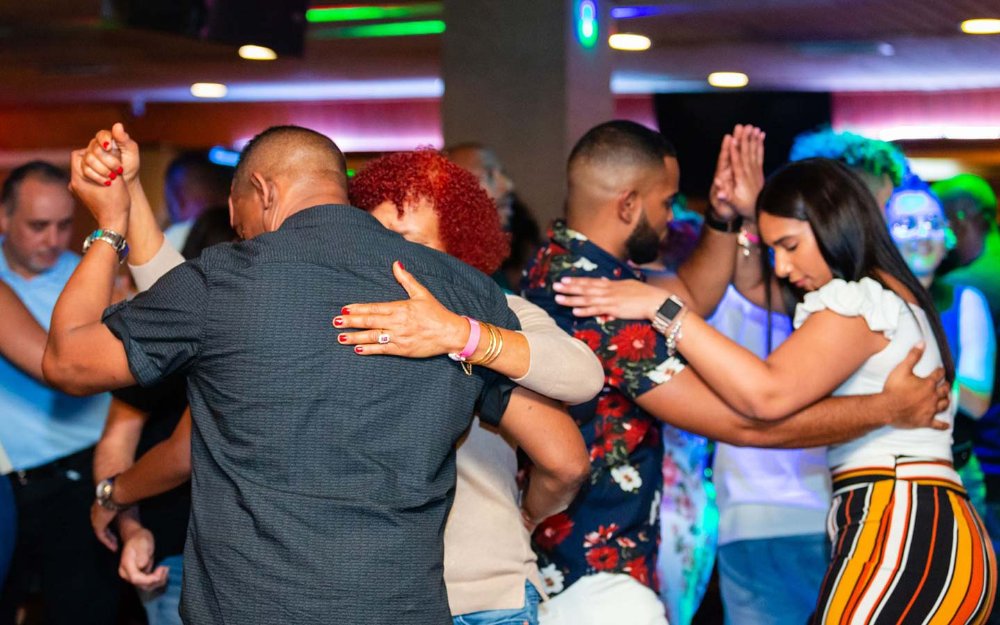The image captures a lively scene in what appears to be a dance hall or club with atmospheric lighting reminiscent of a bowling alley, featuring lively neon colors in pink, purple, blue, and green. The setting is characterized by a low ceiling with various lights not far from the dancers' heads, and a stone support column positioned in the center of the image. 

In the foreground, on the left-hand side, a man with a dark gray, short-sleeved collared shirt stands with his back to the camera, enveloping a woman with short curly red hair in his arms, her face nestled against his shoulder. She wears a cream-colored long-sleeve shirt and jewelry on her wrist. To their right, another couple dances: the man in a blue short-sleeved collared shirt adorned with red flowers and white pants, while the woman wears a white shirt with ruffled sleeves and vibrant striped pants in yellow, orange, white, and black.

The background is slightly out of focus, revealing more people dancing and mingling under the colorful lights, creating a lively and vibrant atmosphere. Multiple light sources illuminate the scene, contributing to the dynamic and festive ambiance, with no visible borders or text on the image.